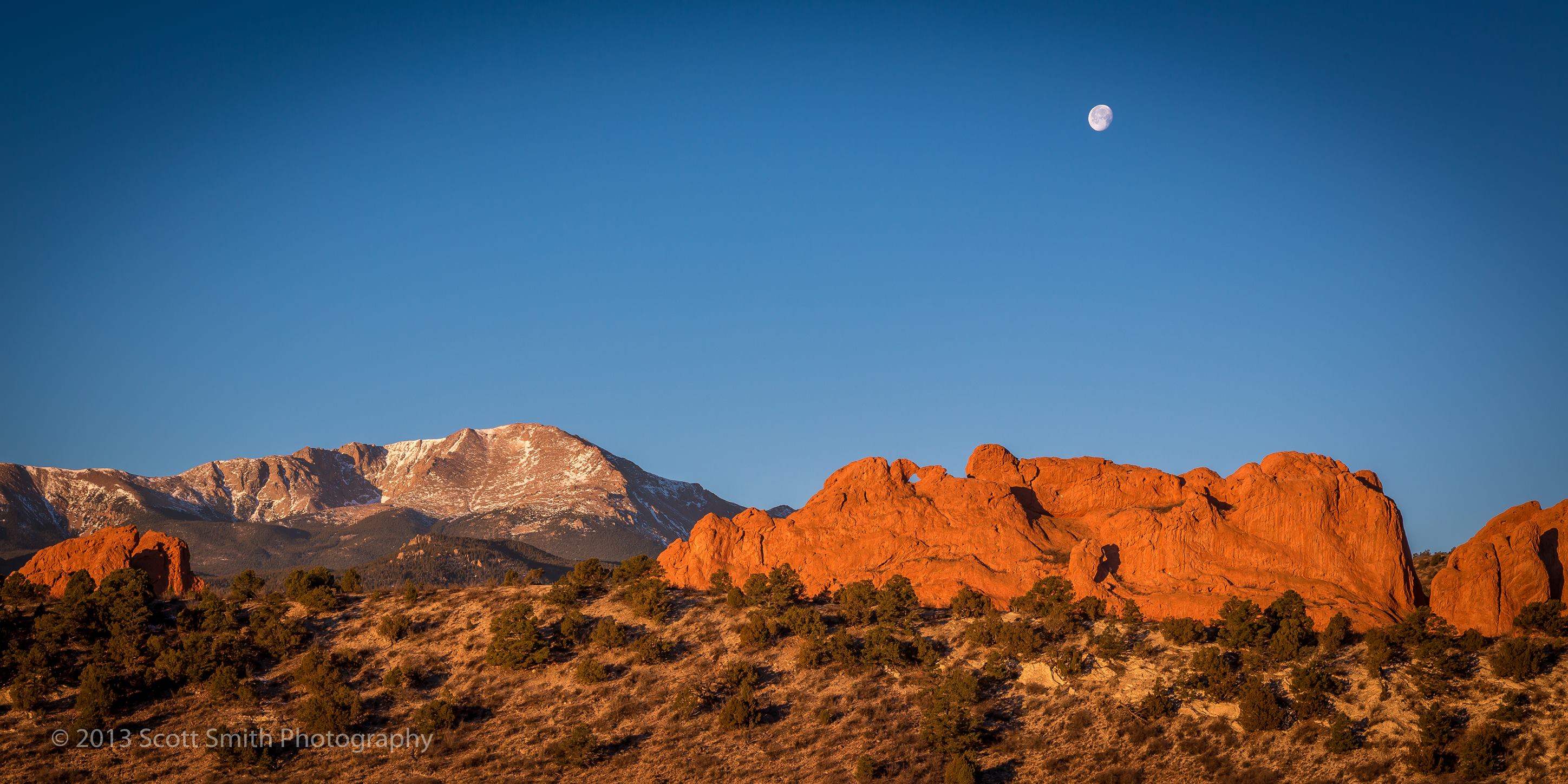This full-color photograph captures a captivating nature scene, likely situated in the American Southwest, during the day under natural light. The lower portion of the image reveals a sandy desert landscape dotted with green vegetation, including small shrubs and trees. Moving towards the middle of the picture, on the right side, there is a striking red rock formation reminiscent of canyon walls, while the left side features a taller, more mountainous terrain, with some areas appearing snow-capped and predominantly light brown. The upper half of the image is dominated by a clear blue sky, devoid of any clouds, highlighting a three-quarter moon positioned in the upper right corner. A subtle white text watermark in the lower left corner reads "Copyright 2013 Scott Smith Photography."